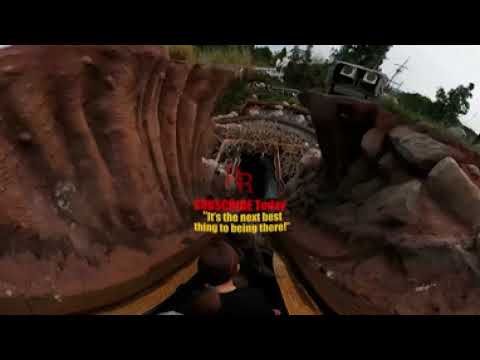The image depicts a ride entering a tunnel, likely at a themed amusement park. In the center, rows of people are visible, seated in what resembles a small boat, hinting at a water-based attraction, possibly Splash Mountain at Disneyland. On the left side of the image, there's a prominent, textured, reddish-brown wall, while the right showcases layered rocky formations with patches of green grass atop. Above the ride, a small building or shack with two windows is nestled into the hill. The sky, visible on the upper right, confirms the outdoor setting. In the middle of the image, bold, yellow text reads, "It's the next best thing to being there!" and above that, in red letters, the text "Subscribe today" is partly visible, indicating this might be a promotion or capture from a video urging viewers to subscribe. The scene is framed with a thick black border on the top and bottom edges.